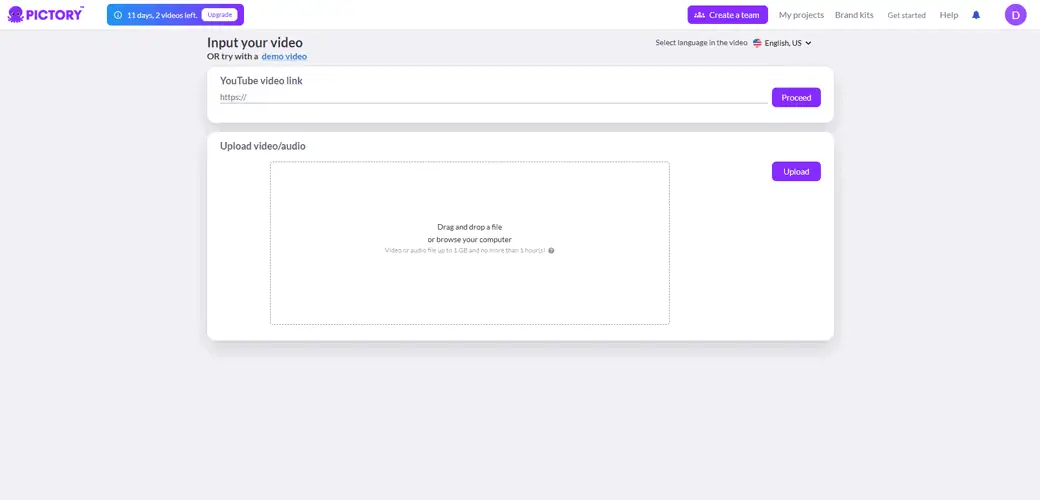The screenshot depicts the interface of a video creation platform named PICTORY. At the top, a white banner prominently displays the PICTORY logo in purple, accompanied by a potential trademark symbol above the brand name. To the right, a purple button indicates a countdown with text partially reading, "11 days, 2 [unreadable] left," alongside a white button labeled for more information.

Further along the banner, another purple button invites users to "CREATE ALBUM" or a similar action. Adjacent to this are navigation options in white text: "MY PRODUCTS," "BRAND KITS," "GET STARTED," and "HELP." The banner also includes a notification bell icon, which shows no alerts, and an ambiguous purple icon resembling either a question mark or a magnifying glass.

Beneath the banner, the interface prompts users with the options "INPUT YOUR VIDEO" or "TRY WITH A DEMO VIDEO," with a selection for video languages defaulting to US English. Users are provided with input fields to enter a video link, along with options to upload video and audio files directly to the platform.